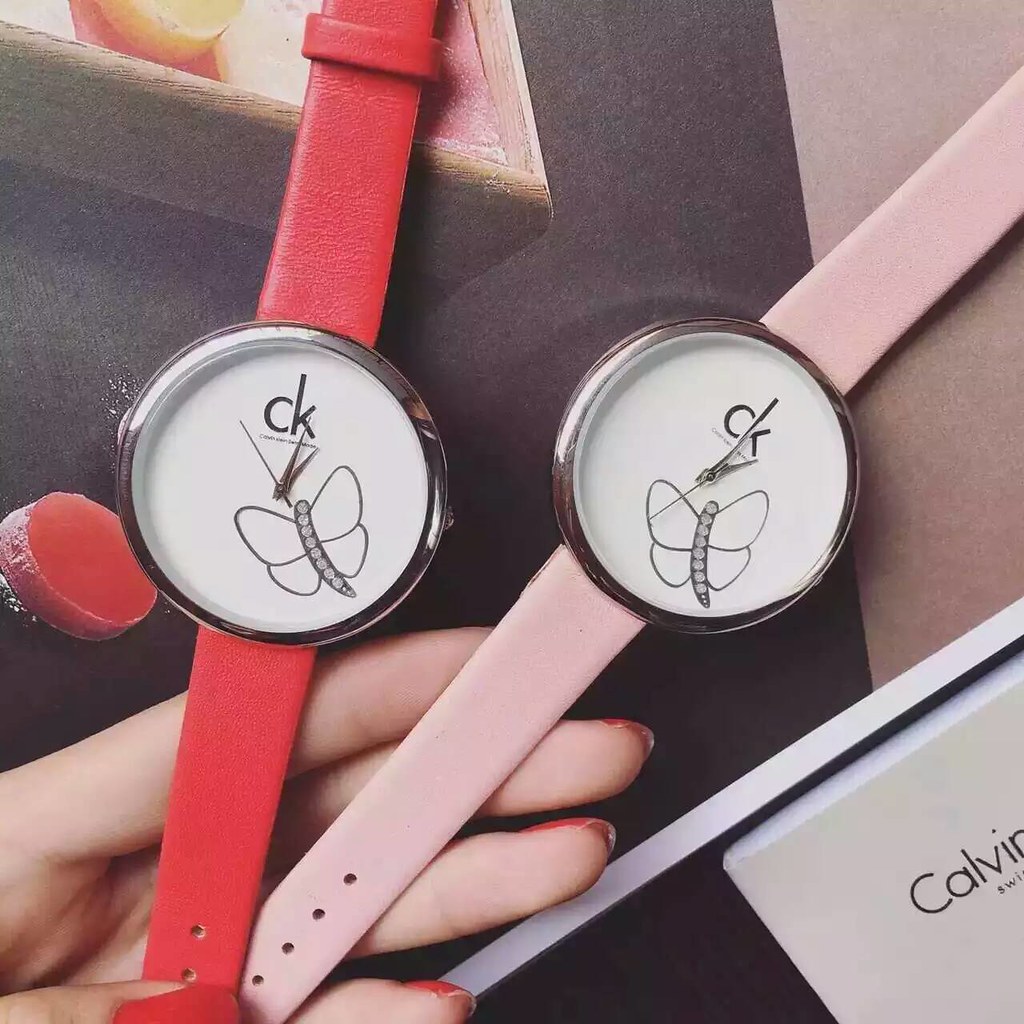This image showcases two elegant Calvin Klein wristwatches, both featuring the iconic CK logo prominently displayed on their faces. Both timepieces share an identical design, characterized by a sleek, silver chrome circle encasing the watch face. A delicate butterfly illustration adorns the face of each watch, embellished with subtle diamond accents along its body, adding a touch of luxury and sophistication. The wristbands differ in color, with one in a striking candy red and the other in a soft pink, both made from supple leather. The model in the photo, with a fair complexion and adorned with dark red nail polish, gently holds the watches, adding a graceful human element to the composition.